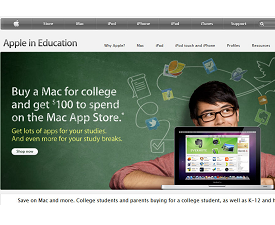The image is a detailed screenshot of a webpage, likely from Apple's website, and is in a landscape orientation with dimensions approximately one-and-a-half times as wide as it is tall. The topmost section features a narrow horizontal gray navigation bar with white font detailing various categories, including the Apple logo on the far left, followed by readable words such as "Home," "iPad," "iPod," and an indistinguishable number of other items, ending with a white magnifying glass icon for search on the right.

Beneath this navigation bar is a lighter gray secondary bar with black font reading "Apple Education," accompanied by several subheadings stretching across to the right. Anchoring the center of the screenshot is an image featuring an Asian man positioned in the bottom right-hand corner, identifiable by his black hair and glasses. He is wearing a red shirt with sleeves rolled up to the elbow and has a laptop open in front of him. The laptop screen displays a mix of green and white elements, framed by a distinctive purple border.

The background behind the man resembles a green-tinged blackboard adorned with various small icons and chalk-like drawings. To the left of the central image, white text reads: "Buy a Mac for college and get $100 to spend on the Mac App Store." Below this, in yellow, it states: "Get lots of apps for your studies, and even more for your study breaks."